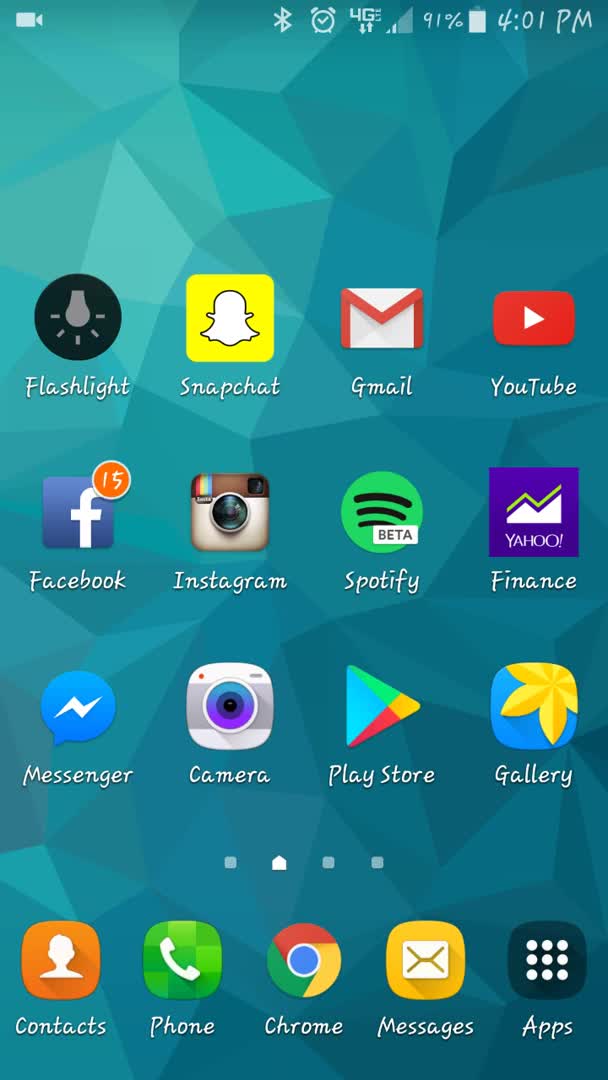The image depicts a smartphone interface which appears to be an Android device, given the presence of the Google Play Store icon. The background is a turquoise color with a crystalline or geometric pattern, adding a modern and vibrant aesthetic. 

At the top of the screen, a row of status icons indicates various device conditions: there is ongoing recording, Bluetooth is enabled, an alarm is set, the device is connected to a 4G LTE network with two bars of signal strength, the battery is at 91%, and the time is 4:01 p.m. The standard font has been customized to an informal, handwritten style, imparting a personalized touch to the device's interface.

The layout of the app icons is organized into several rows:
- The top row includes the Flashlight, Snapchat, Gmail, and YouTube icons. The Flashlight is depicted as a round black circle with a glowing gray light bulb, while the other icons are the standard ones associated with their respective apps.
- The second row contains Facebook, Instagram, Spotify, and Yahoo Finance. Notably, the Facebook icon displays a notification count of 15. The Yahoo Finance icon features a line graph superimposed on a blue background with the text "Yahoo".
- The third row features Messenger, Camera, Play Store, and Gallery icons. The presence of the Play Store icon confirms the device is running on an Android operating system.
- The final row includes Contacts, Phone, Chrome, Messages, and Apps icons.

Each app icon is easily recognizable by its standard design, except for the customized Flashlight icon, enhancing the overall usability of the device. The detailed array of app icons and status indicators provides a comprehensive overview of the smartphone's functionalities and current status.